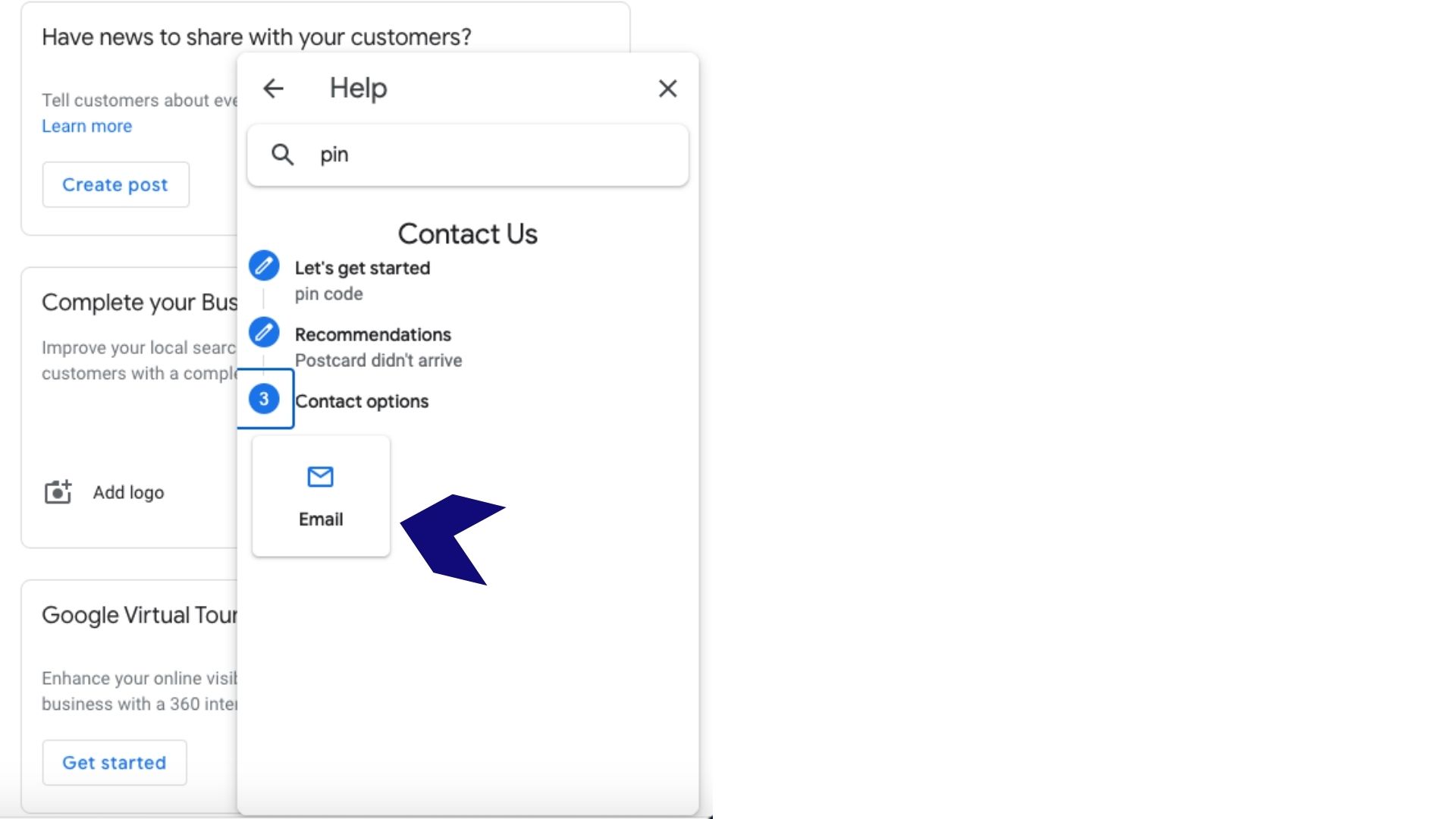The image is a detailed screenshot of a website's Help Center interface. At the top left corner, there's a bold statement reading "Have news to share with your customers." Adjacent to this, on the right, a pop-up window labeled "Help" is prominently displayed. In the center of this window is a search box with the word "PIN" inside it. Below the search box, prominently featured, is a "Contact Us" option. To the left, there's a list of links under the heading "Let's Get Started." The links include "PIN Code," "Recommendations," "Postcard Didn't Arrive," and at the bottom, "Contact Options" with a specific choice for "Email."